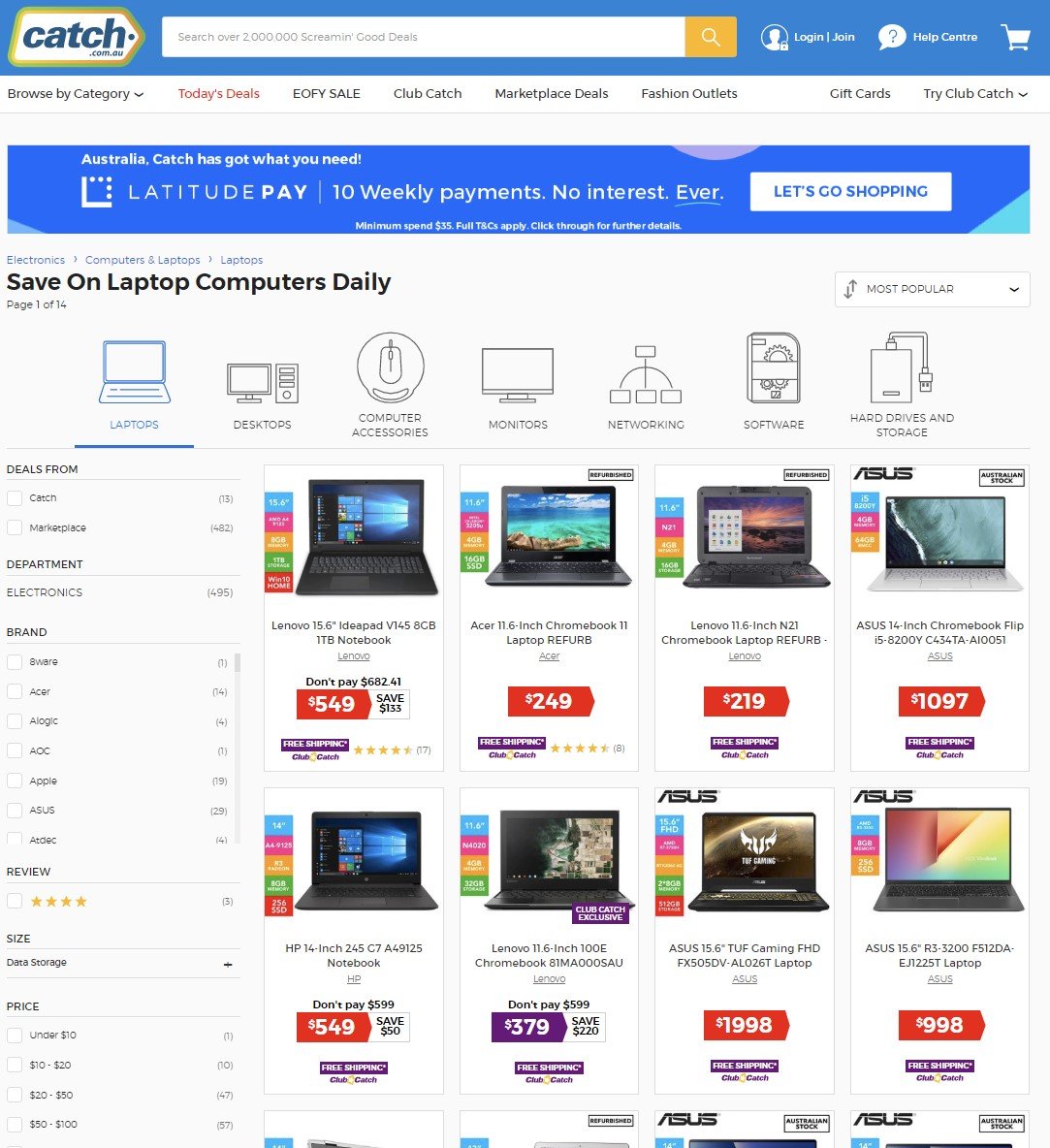This is a detail-rich description of Catch's website interface:

The website of Catch features the company's logo prominently in the upper left-hand corner, resembling a tag with blue text. Adjacent to the logo, a search bar is available for ease of navigation, accompanied by options to log in, join the platform, access the help center, and view the shopping cart.

Directly beneath these elements, a navigation bar highlights several categories such as "Browse by Category," "Today's Deals" in red, "Sale," "Club Catch," "Marketplace Deals," "Fashion Outlets," "Gift Cards," and "Try Club Catch." Below this, a blue bar spans the website's width, displaying important promotional information: "Australia, Latitude Pay, ten weekly payments, no interest ever."

The next section promotes savings on laptop computers with a banner that reads "Save on Laptop Computers Daily." This banner is highlighted with appealing imagery and pricing details, organized into two rows of laptop images. Each laptop listing features its price prominently on a red ticket. The laptops are from various reputable brands, including Asus, Lenovo, and HP, with a standout deal highlighted in purple, offering a laptop for $379.

On the left side of the webpage, users can filter their search based on preferences for laptops, desktops, monitors, networking equipment, software, and hard drives, facilitating a tailored shopping experience.